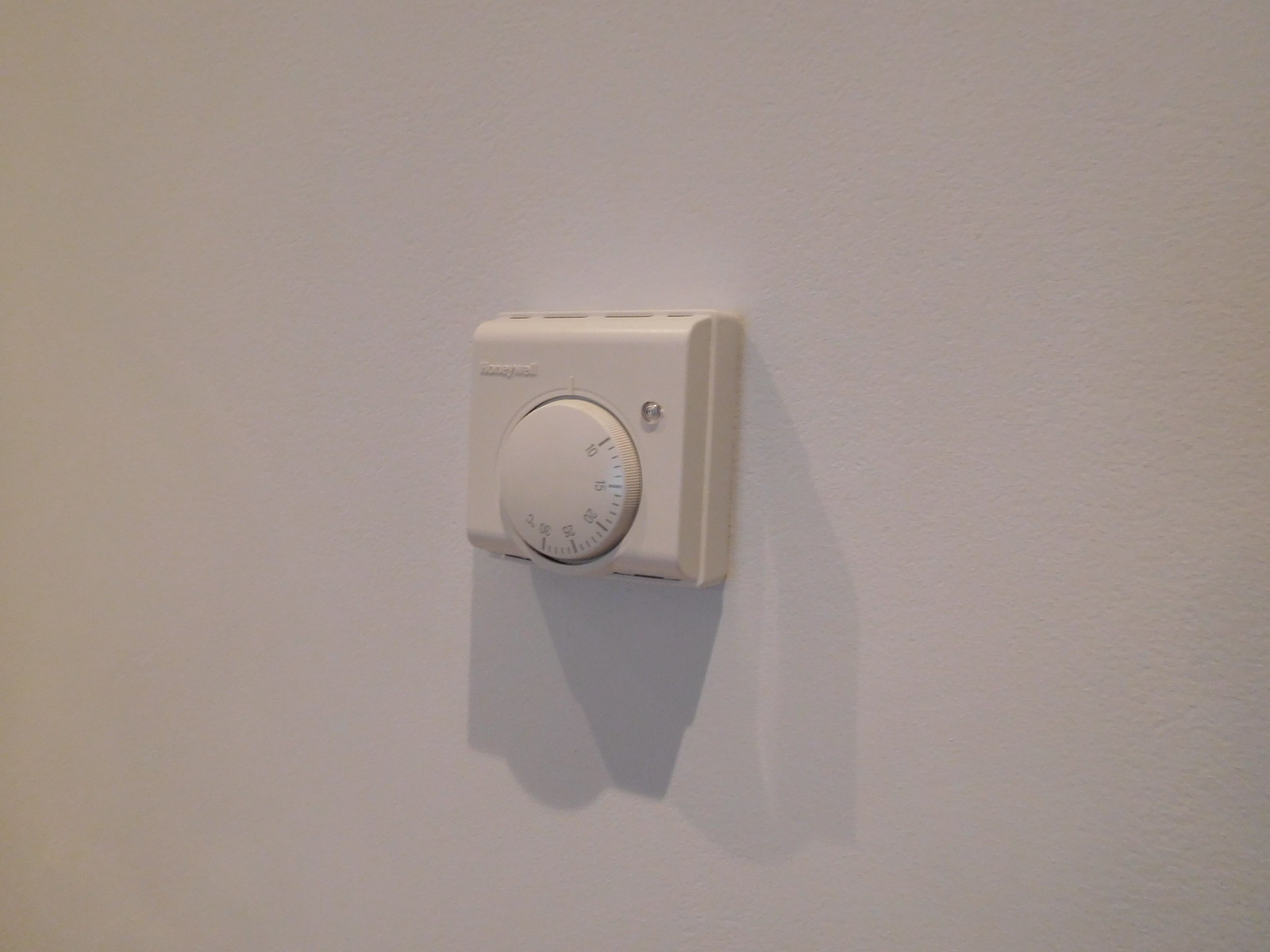This color photograph features a close-up of a Honeywell thermostat mounted on a slightly textured beige wall. The thermostat is centered in the frame, captured from a slightly diagonal, sideways angle. The thermostat itself is also beige and is square in shape with a large, circular dial prominently placed in the middle. The dial, which ranges from 10 to 30 degrees Celsius with intermediate markings at 15, 20, and 25 degrees, is encircled by a lined texture which adds to the visual detail. The brand name "Honeywell" is visible in the upper left corner of the thermostat. A shadow cast by light above falls beneath the device, adding depth to the image. The wall around the thermostat is bare, further emphasizing the focus on the object.